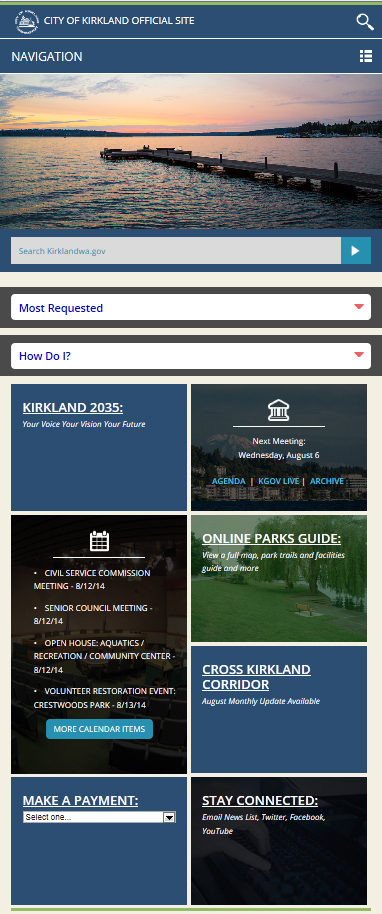In this image, we see the official website of the City of Kirkland. The top of the webpage displays the header "City of Kirkland Official Site" along with a navigation menu and a magnifying glass icon for search functionality. Below the header, there's a picturesque photograph of a dock extending into the ocean against the backdrop of a stunning sunset.

The central section of the webpage features a search field labeled "Search KirklandWA.gov" and several prominent sections, including "Most Requested," "How do I?" and "Kirkland 2035: Your Voice, Your Vision, Your Future." Information about upcoming events is also listed, such as the next meeting on Wednesday, August 6th, with details on the agenda including 'K-Gov Life Archive,' the Civil Service Commission meeting scheduled for August 12th, 2014, and the Senior Council meeting on the same date. There's also an announcement for an open house event on aquatics and the recreation community center, and information regarding a Volunteer Restoration event at Crestwood Park, taking place on August 13th, 2014.